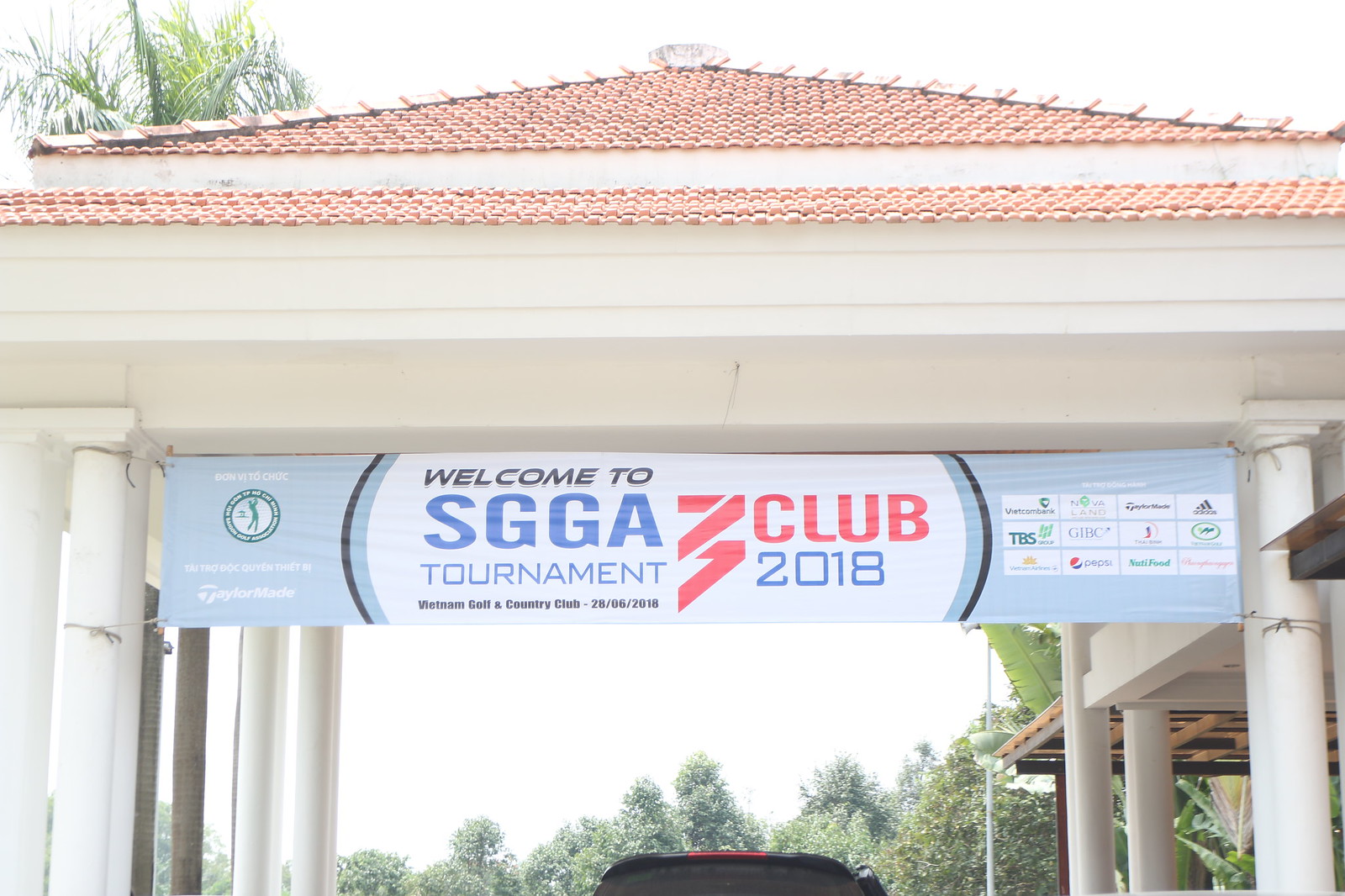The photograph captures an outdoor setting featuring a striking, multi-layered archway with an oriental-inspired design. The archway includes white posts and cross beams holding up a dual-level roof; the top level features an orange terracotta tile roof while the lower level has a smooth, white surface that tapers down to its edge. This structure resembles the kind of covered drive-through area typically found at hotels or resorts.

Prominently displayed beneath the roof is a large banner. The banner is divided into three sections. The left third has a light blue background with the image of a golfer finishing his shot and a black border separating it from the central section. The middle segment reads "Welcome to SGGA Tournament" in bold black and blue text, followed by "Vietnam Golf and Country Club, 26-06-2018." The right portion of the banner features red symbols resembling two 'V's, flanked by a series of twelve small sponsor logos, some recognizable such as Pepsi, Adidas, TBS Group, Vietcom Bank, Novaland, and NutriFood.

Beneath this banner, you can see the top of a black car with a red stripe and dark tinted windows. The surroundings behind the structure show a hazy blue sky with floating, indistinct clouds and a line of leafy green trees, adding a serene backdrop to the scene.